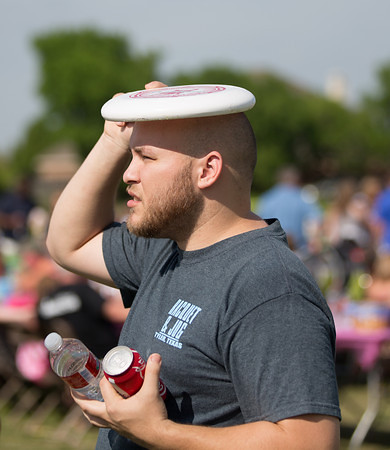In the image, we see a young man with a bald or closely shaven head and a short, dark beard, standing outside on a sunny day. He is wearing a short-sleeved gray t-shirt that has some white writing across the left chest area, though the text is mostly indecipherable. Utilizing his right hand, he holds a white frisbee with a red design over his head to shield himself from the bright sun. His left hand carries a clear plastic water bottle and a can of Coca-Cola. The man, who appears muscular and slightly larger in build, is squinting and looking left, with his mouth slightly open, revealing a glimpse of his teeth. The background is blurry but shows multiple people, likely spectators, and lush green trees under a grayish-blue sky, indicating a daytime outdoor event.